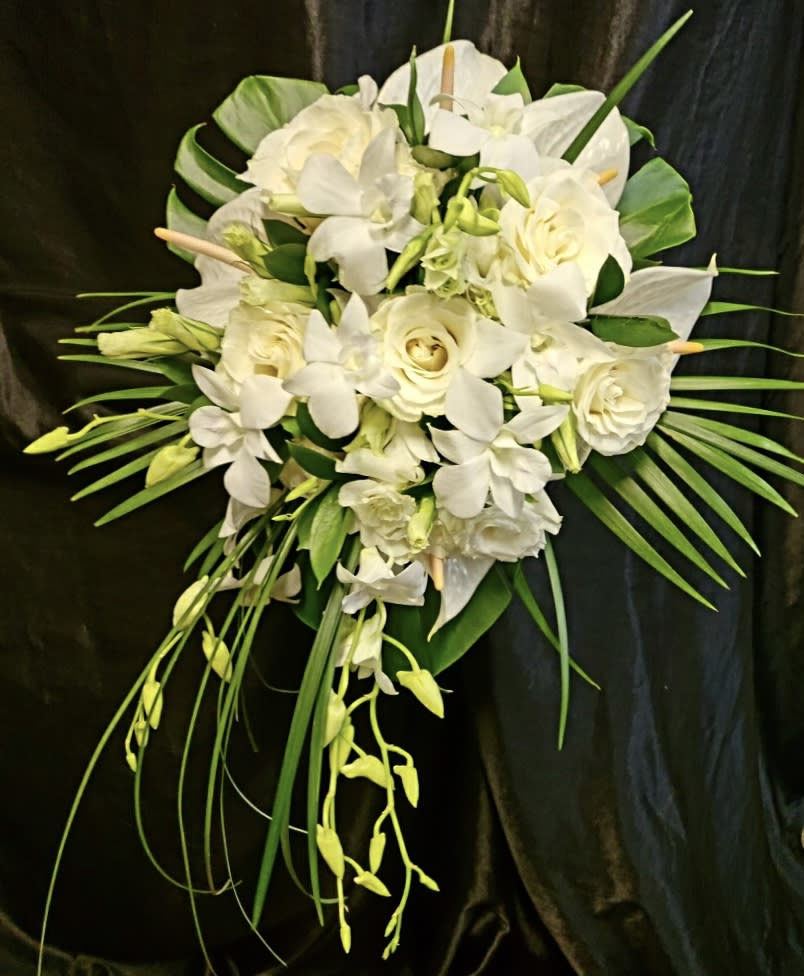The photograph features a lush bouquet of white flowers, primarily white roses, nestled in vibrant greenery. The bouquet, nearly heart-shaped, contains additional white lilies and other delicate white blossoms, interspersed amidst the roses. Long, frond-like green leaves and sword-like blades surround the flowers, while a few tendrils and vines with unblossomed buds cascade downwards. Some green spikes and broad leaves are also visible at the top of the arrangement. The background showcases a dark, umber-colored satin drape, adding a rich, textured backdrop that contrasts with the bright lighting on the white flowers. This creates an almost ethereal appearance, making the bouquet seem as if it is floating in mid-air.